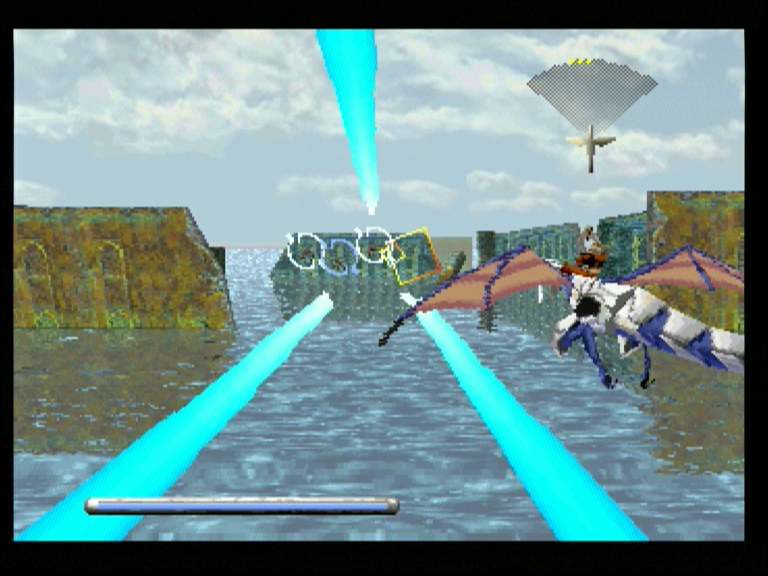This is a screenshot from a Sega Saturn game, likely either "Panzer Dragoon" or "Panzer Dragoon II." The image has a distinct retro aesthetic, with a black border framing the pixelated landscape. Dominating the background is a very cloudy and generated sky filled with white clouds. The landscape features square-looking "mountains" in various shades of green and gray. In the foreground on the right, a blue and white dragon with a rider wearing a light-colored top can be seen flying.

In the upper right section, there is a darker HUD element with a small image that resembles a bird, though it’s not exactly clear. Bright blue beams of light stretch across the middle of the screen, giving a dynamic sense of action. The background also contains white and purple shapes highlighting unseen enemies. Turquoise lines in the foreground suggest perspective lines leading towards possible water or stone structures. At the bottom left, there's a long silver rectangle which likely represents a full health bar. The overall scene is vibrant yet intricate, capturing the essence of classic video game design.